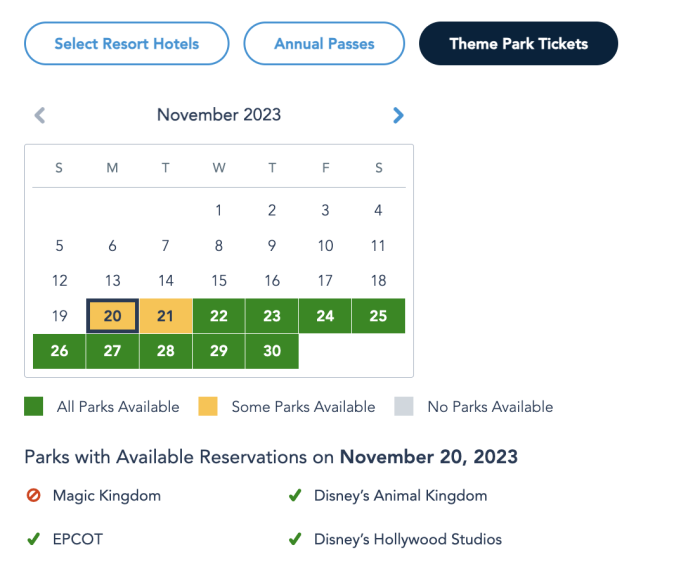The image displays a Disney reservation interface that could be accessed on either a desktop or a mobile device. The interface allows users to select tickets or passes for various Disney attractions. At the top of the screen, there are three selectable bubbles labeled "Resort Hotels," "Annual Passes," and "Theme Park Tickets," with "Theme Park Tickets" currently selected. 

Below these options, a calendar interface is displayed, allowing users to toggle through dates. The specific calendar shown is for November 2023, highlighting dates from Monday, November 20th, to Thursday, November 30th. On November 20th and 21st, only some parks are available, indicated in yellow. From November 22nd to 30th, all parks are available and highlighted in green.

The specific date of November 20th is selected, and the bottom portion of the screen shows "Parks with Available Reservations on November 20th, 2023." Here, it indicates that Magic Kingdom is unavailable, denoted by a red stop symbol. In contrast, Epcot, Disney's Animal Kingdom, and Disney's Hollywood Studios all have available reservations, marked with green checkmarks beside their names.